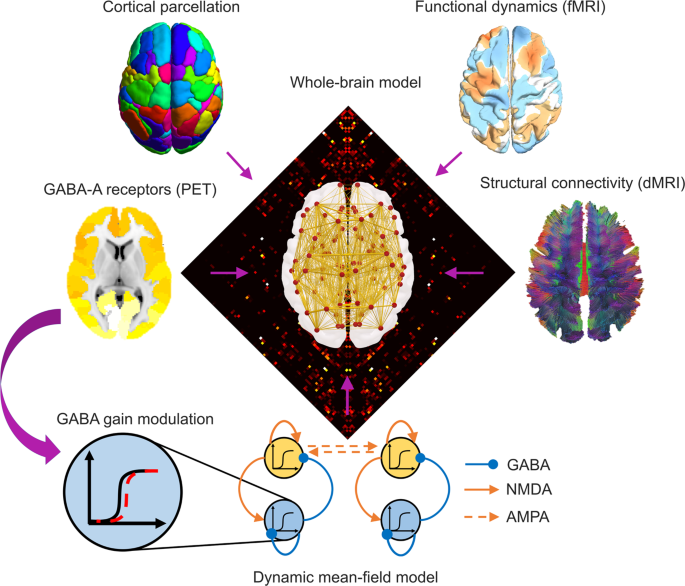The detailed diagram showcases a central "whole brain model" set against a diamond-shaped black background. Within this main image, the left and right hemispheres of a brain are outlined in white, interwoven with crisscrossing yellow lines and intersecting red dots, symbolizing neural connections. Surrounding the central brain image are smaller, color-coded brain diagrams connected by purple arrows. Each of these peripheral diagrams represents different aspects of brain function and anatomy, labeled as: "cortical parcellation" portrayed with a colorful, play-doh-like appearance; "functional dynamics (fMRI)" in shades of white, brown, and blue; "GABA-A receptors (PET)" featuring a yellow brain with a white interior; and "structural connectivity (dMRI)" depicted with pink, purple, and green stripes. Additionally, there is a specialized inset on the left indicating "GABA-A gain modulation," with a blue circle and detailed illustrations, labeled "GABA-MNDA and AMPA" and associated with the "dynamic mean field model." The entire graphic, set on a plain white background, measures approximately four to five inches square. At the top, the title "whole brain model" is prominently displayed in black print.